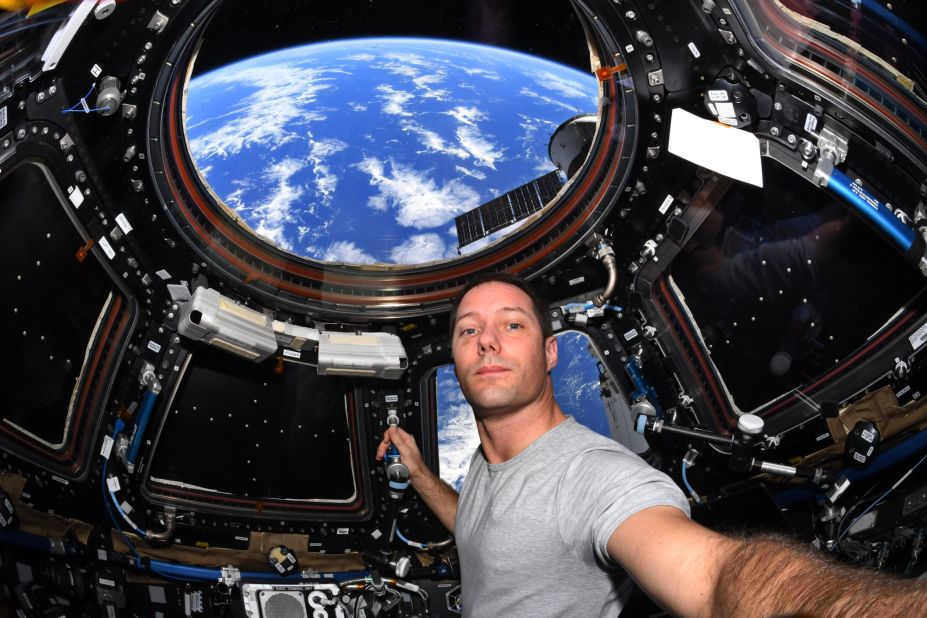In the selfie picture, a white male with dark hair and blue eyes can be seen wearing a light gray t-shirt. He is extending his left arm to take the selfie, while his other hand holds an unspecified object. The man is situated inside a space shuttle or satellite. The interior of the spaceship features numerous controls, both silver and black buttons, and is marked by blue and white wires. Surrounding walls are lined with black panels, which might be screens, and there are three square windows visible. Through a circular window at the top, the Earth is visible against the black backdrop of space, adorned with white stars. The Earth appears blue with white clouds, and part of a satellite can also be seen through one of the windows.